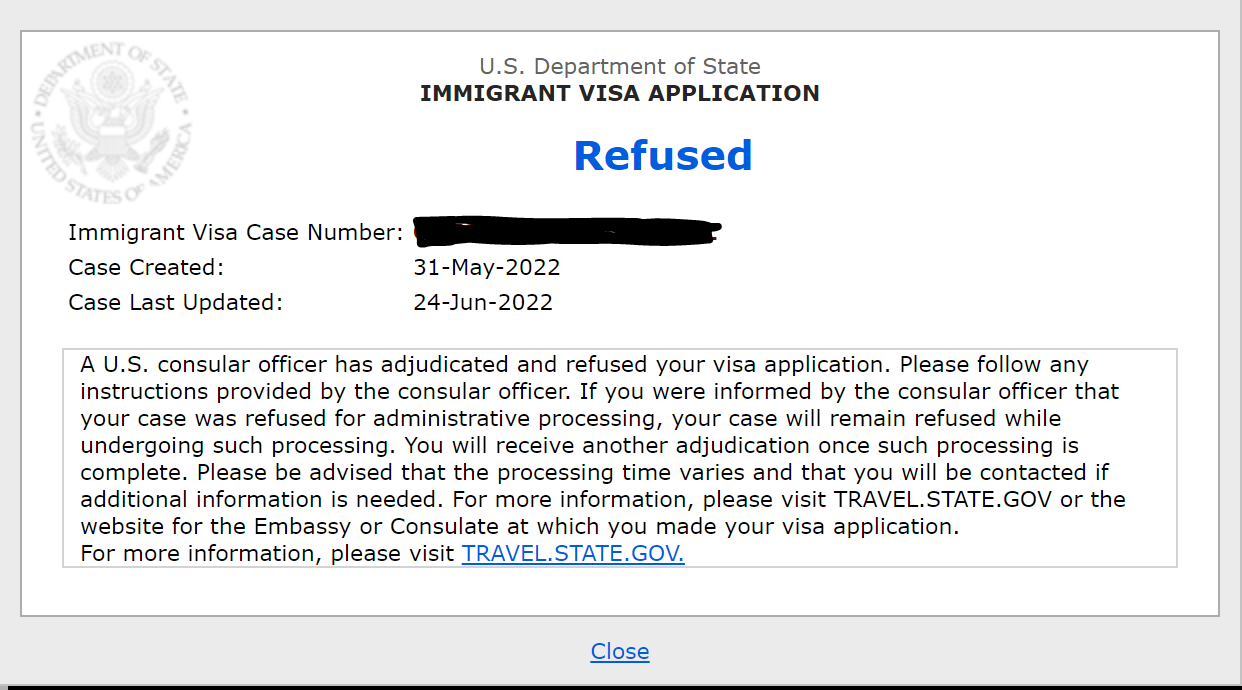**Caption:**

A screenshot featuring a gray background and a prominent white box. On the left side of the box, there is text indicating "US Department of State Immigrant Visa Application" and a blue "Refused" status. Below this, blacked-out text conceals the specific immigrant visa case number. The case was created on May 31, 2022, and last updated on June 24, 2022. It states that a U.S. consular officer has adjudicated and subsequently refused the visa application. The notice instructs the applicant to follow any provided guidance from the consular officer. It also mentions that if the refusal is due to administrative processing, the case will remain refused during this period. A subsequent adjudication will be issued once processing is finalized. The processing time can vary, and the applicant will be contacted if additional information is required. For further details, the notice directs readers to visit travel.state.gov or the website for the specific U.S. embassy or consulate where the visa application was submitted.